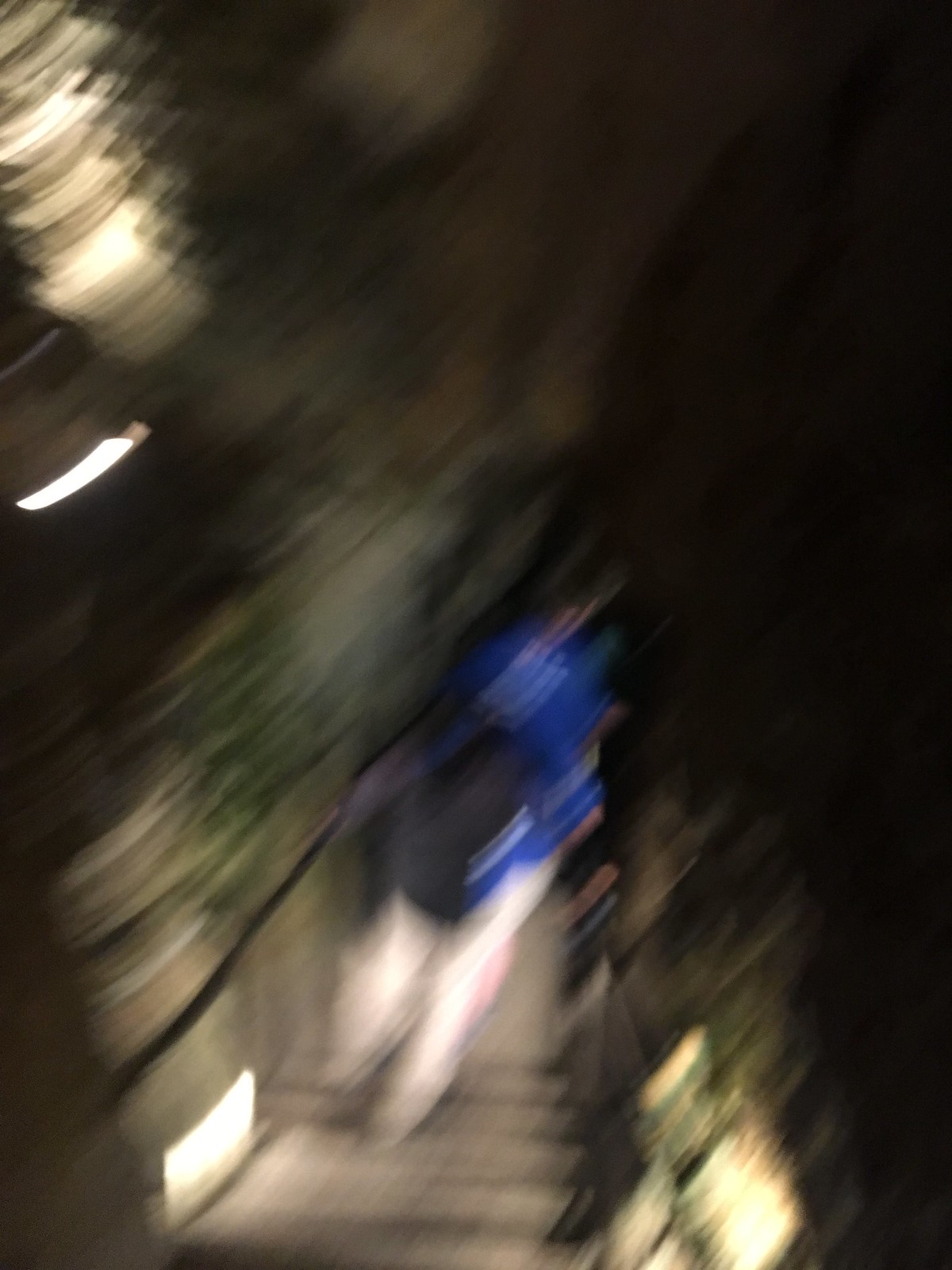A person, likely female, is descending a staircase with an iron railing. She has brown hair and is wearing a blue shirt paired with white pants. She carries a black backpack and holds a pink item, possibly a bag, in one hand. In her other hand, she holds a long object, perhaps a yoga mat, while looking down attentively at something in front of her. The background is blurry, featuring a mix of green, brown, and tan colors.